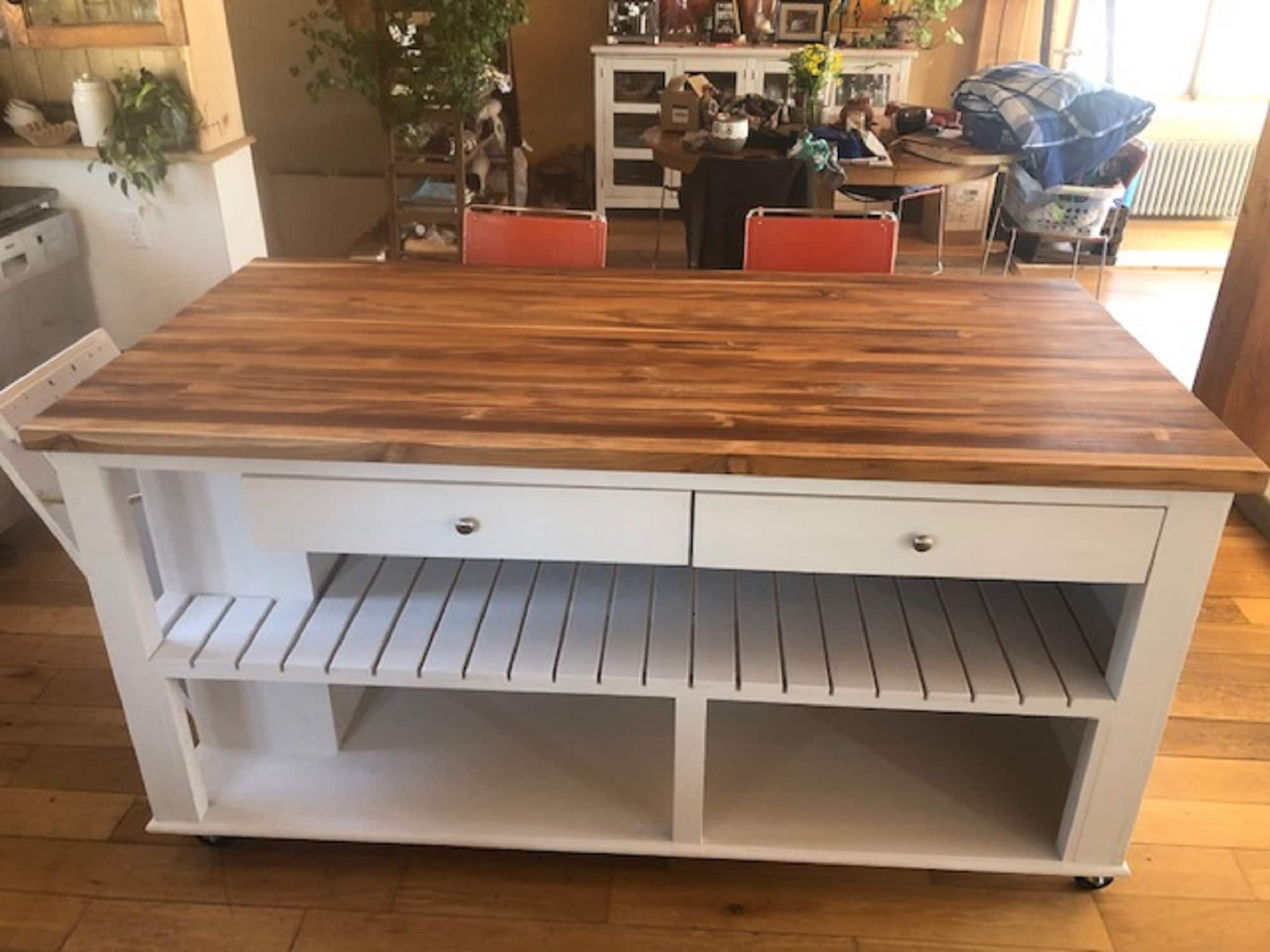This is a detailed photograph of a multifunctional kitchen-dining area in what appears to be a residential setting. The central focus is a mobile kitchen island situated slightly to the right of the image. The island is mainly white with a brown wooden tabletop showcasing distinct wood grain. It features two drawers at the front, an open slatted wood shelf below, and an additional open storage space at the bottom. Flanking the island are three chairs—one white chair on the left and two red chairs in the middle. 

To the left of the island, there's a partially open door that appears to be part of built-in storage or an appliance like a dishwasher. The background reveals more of the room; there is another table cluttered with various household items, indicating a lived-in environment or ongoing packing/unpacking activities. At the far end, a sideboard houses photo frames and indoor plants, contributing to the cozy and personalized atmosphere. The floor is also wooden, blending seamlessly with the island's wooden tabletop and contributing to the warmth of the space.